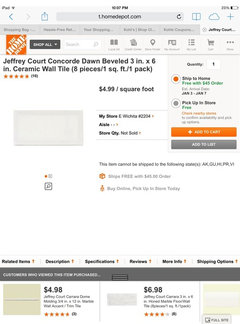A screenshot from HomeDepot.com is displayed on a tablet using the Safari browser. The interface looks slightly larger than a phone view but still maintains a mobile-friendly ratio. The specific webpage features a product listing for the Geoffrey Court Concord Dawn beveled 3-inch by 6-inch ceramic wall tile. The image of the tile is small but shows a beige-colored ceramic tile. The cost is noted as $5 per square foot, with each pack containing 8 pieces. The page shows checkout options, and the user has chosen the "ship to home" option, which is selected over the "pick up" option. Though the text is small and hard to read, additional recommendations are visible at the bottom of the screen, showing other tiles priced at around $7 each. The selected product boasts 5-star reviews.